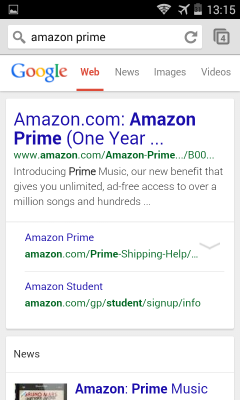The screenshot appears to be taken from an Android device. In the upper-right corner, the Wi-Fi icon shows a full three-bar signal strength. However, there seems to be an unusual vertical line running from top to bottom through the Wi-Fi icon, possibly indicating a malfunction. Next to the Wi-Fi icon, the airplane mode is activated, and the battery level icon, without a percentage but visibly low, seems to indicate it is at approximately 18%. The time displayed is 13:15. 

Below the status bar, a search input field is visible with a magnifying glass icon on the left and a refresh button on the right. The tab is titled "Amazon Prime" with the number of open tabs indicated as 4, positioned just right of the refresh button. Below that is the Google logo followed by four tabs: "Web" (selected and underlined in red), "News," "Images," and "Videos."

In the main body of the screenshot, the text "Amazon.com - Amazon Prime - One Year" is prominently displayed, followed by a green hyperlink, "www.amazon.com/amazon-prime." The text introduces "Prime Music," describing it as a new benefit that offers unlimited ad-free access to over a million songs and hundreds more. Following this, there is a mention of "Amazon Prime" and "Amazon Student," with a drop-down menu available for Prime. At the very bottom, there's a news section titled "Amazon Prime Music."